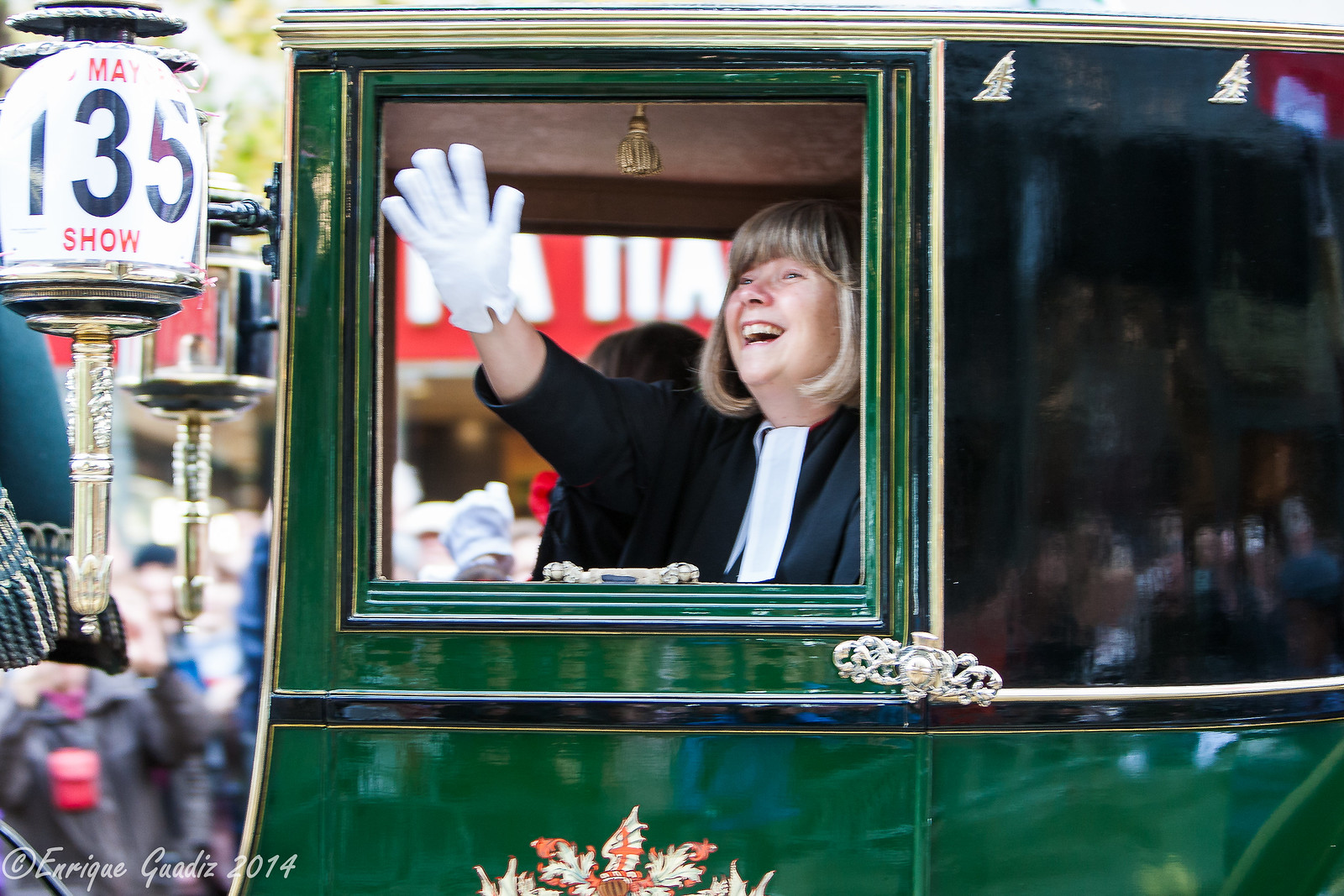This detailed photograph captures a joyous moment of a woman participating in a parade or car show, seated in a distinctively green motorcade. The woman, with short blonde hair and bangs, is dressed in a black gown underneath a white undershirt and is waving brightly with a white-gloved hand. She appears to be seated in a green vehicle that looks a bit boxed, accentuating her cheerful gesture through the open window. The vehicle's side, just below her, features an emblem partially showing a mast with a red cross, hinting at the flag of England. The scene is accentuated by lanterns with gold bases and white flowers with pink tips adorning the top of the carriage. A sign to the left reads "Show" in blue lettering, while the bottom left corner of the photograph is marked with the text “@Enrique Guadiz 2014.”